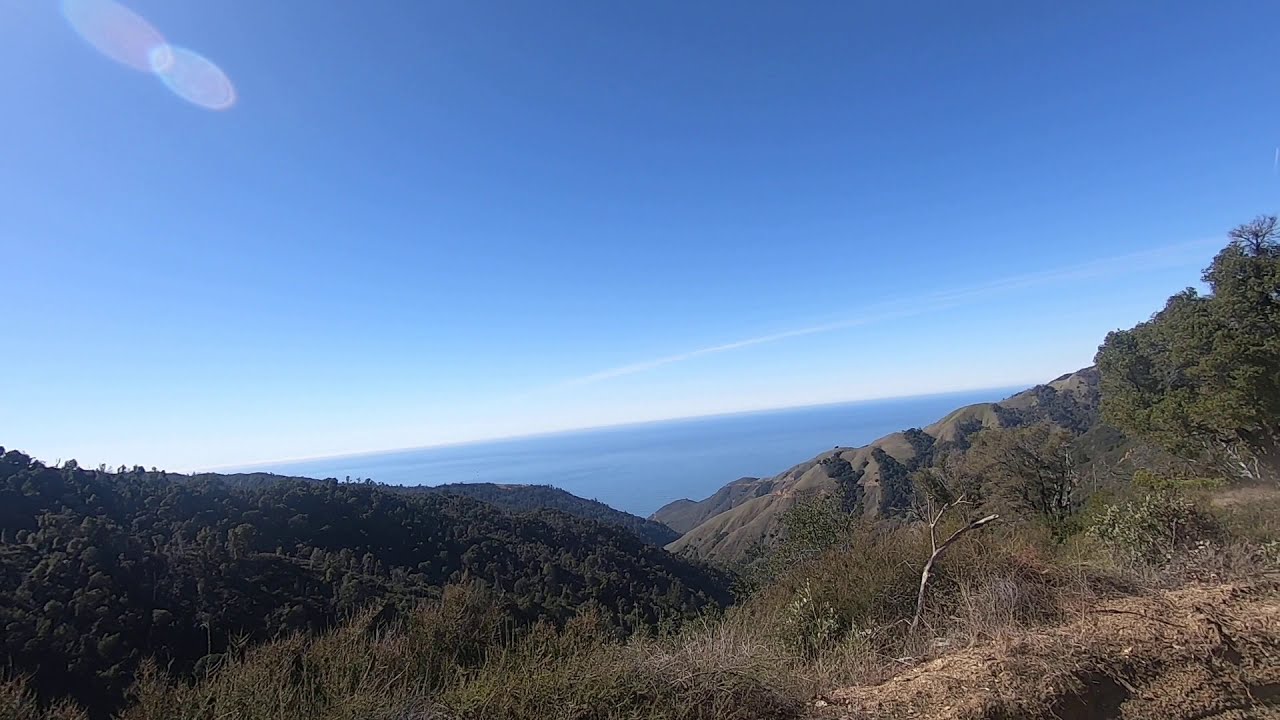In this detailed landscape photograph taken on a bright, clear sunny day with a vivid blue sky, the scene presents a diverse natural environment. The horizon appears to feature a low bank of clouds or possibly the ocean, creating a bright line of white light against the sky. The landscape is characterized by rolling hills forming a wide V shape. The hills on the right are rocky and barren, displaying shades of brown with sparse vegetation, while the hills to the left are lush, covered with dark green trees and shrubs. In the foreground, the terrain is dry and scrubby, dotted with brown bushes and weeds, and a large leafy tree stands off to the right. There are also wispy streaks of white clouds or potentially the trail from a jet plane, adding subtle details to the otherwise clear blue sky. The overall scene conveys a high elevation viewpoint, looking over expansive grasslands and rocky outcroppings towards what might be the distant ocean, enhancing the sense of vast, open space.